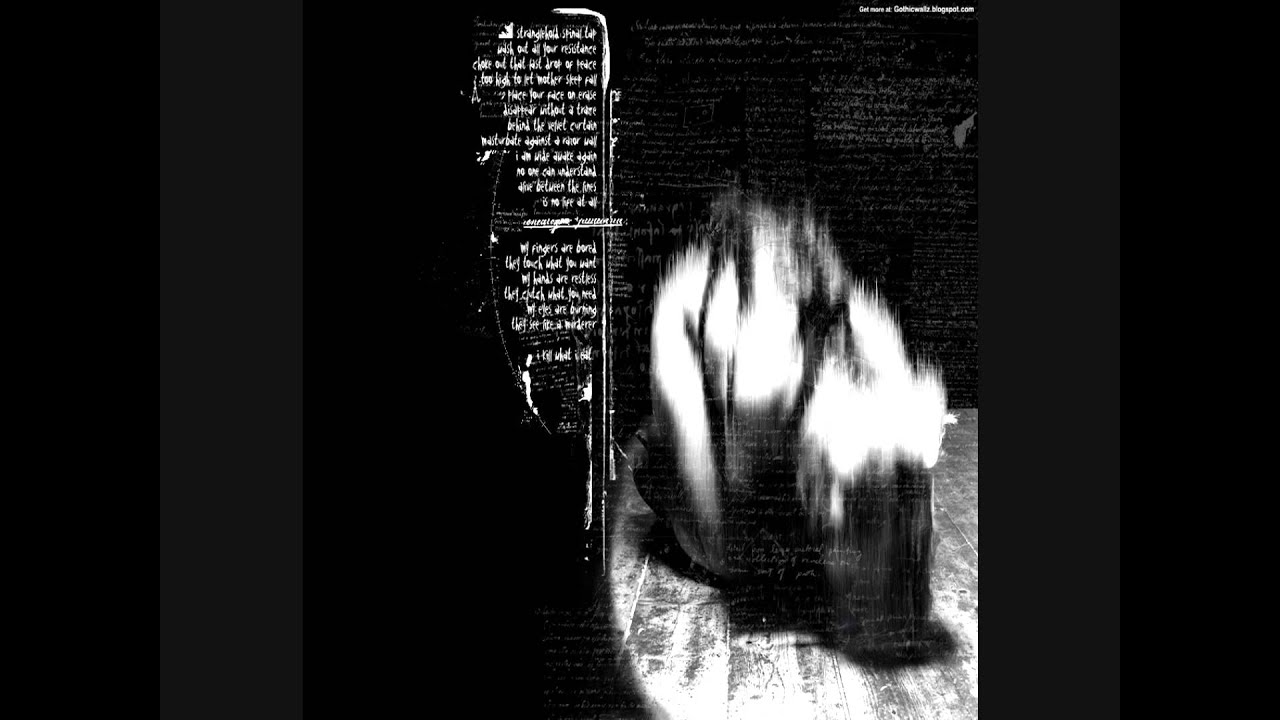This image appears to be an album cover or a page of song lyrics set against a predominantly black background. Central to the composition is a rectangular, black and white distorted photograph of what seems to be a person kneeling on a wood floor. This photograph is bordered by two black edges and also a larger grey background. The top of the object within the photo features some glowing elements, which could be interpreted as lit candles. There is a transparent overlay of writing in the background that adds a textual texture to the image.

On the left side of the composition, there are two paragraphs of white writing, likely song lyrics or a description, separated from the main image by a distinct long white chalky line. The white writing appears small and unreadable but is integral to the overall design. In the top right corner of the image, additional small white text catches the eye. The overall aesthetic gives the impression of a detailed, layered visual experience combining text and imagery on a black background with subtle variations in texture and tone.